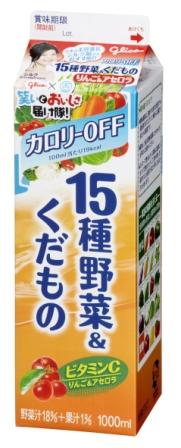A vibrant, quart-sized carton, resembling a common U.S. milk container, stands unopened with its neat, folded cardboard top still intact. The carton is adorned with a blend of oriental characters and sporadic English words, prominently displaying "15" followed by a mixture of foreign and English letters. The base color is a warm orange, extending about two-thirds up the carton, interspersed with some blue lettering. A green leaf with potentially red tomatoes or cherries rests on one side, adding to the colorful design. Along another side, various vegetables are pictured, including tomatoes, carrots, squash, radishes, onions, and peas. Additionally, there are small beads illustrated, suggesting an array of ingredients within this mysterious drink.